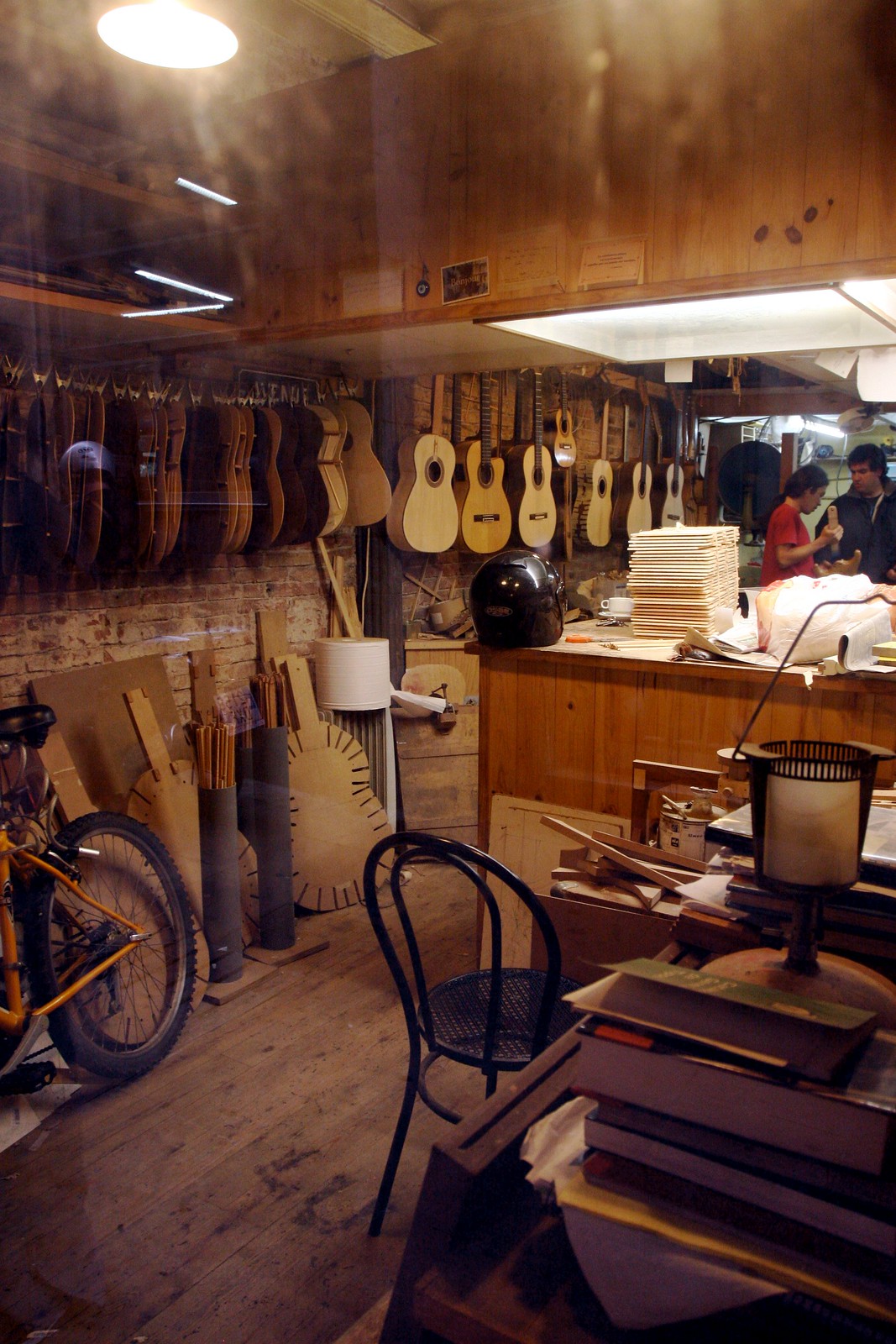The image depicts the detailed interior of a guitar maker's workshop, bathed in mid-day light. The wooden floor sets the base for an assortment of objects and activities that enhance the musical ambiance. To the left, there's a neatly arranged desk with books, tools, and materials typically used for guitar crafting. A black chair is positioned in front of it, inviting one to sit and work. Nearby, a road bike leans against the wall, adding a touch of casual presence to the scene.

At the center of the activity, two individuals are engaged in conversation, possibly discussing guitar craftsmanship. Their lively discussion gives life to the setting. The walls are adorned with framed sketches and various guitars—some unfinished, others ready for sale. The hanging guitars, particularly six completed ones, exhibit intricate markings and polished bodies, exemplifying the intricate work done in this shop.

On the right side of the desk, carvings and components of guitars await assembly, showcasing different stages of guitar-making. A lamp with a wooden stand and a black net top adds to the cozy workshop atmosphere. The diverse palette of browns, tans, blacks, oranges, yellows, reds, greens, and light blues enriches the environment, making the space both vibrant and welcoming. This detailed and immersive setting highlights the meticulous artistry involved in guitar crafting.